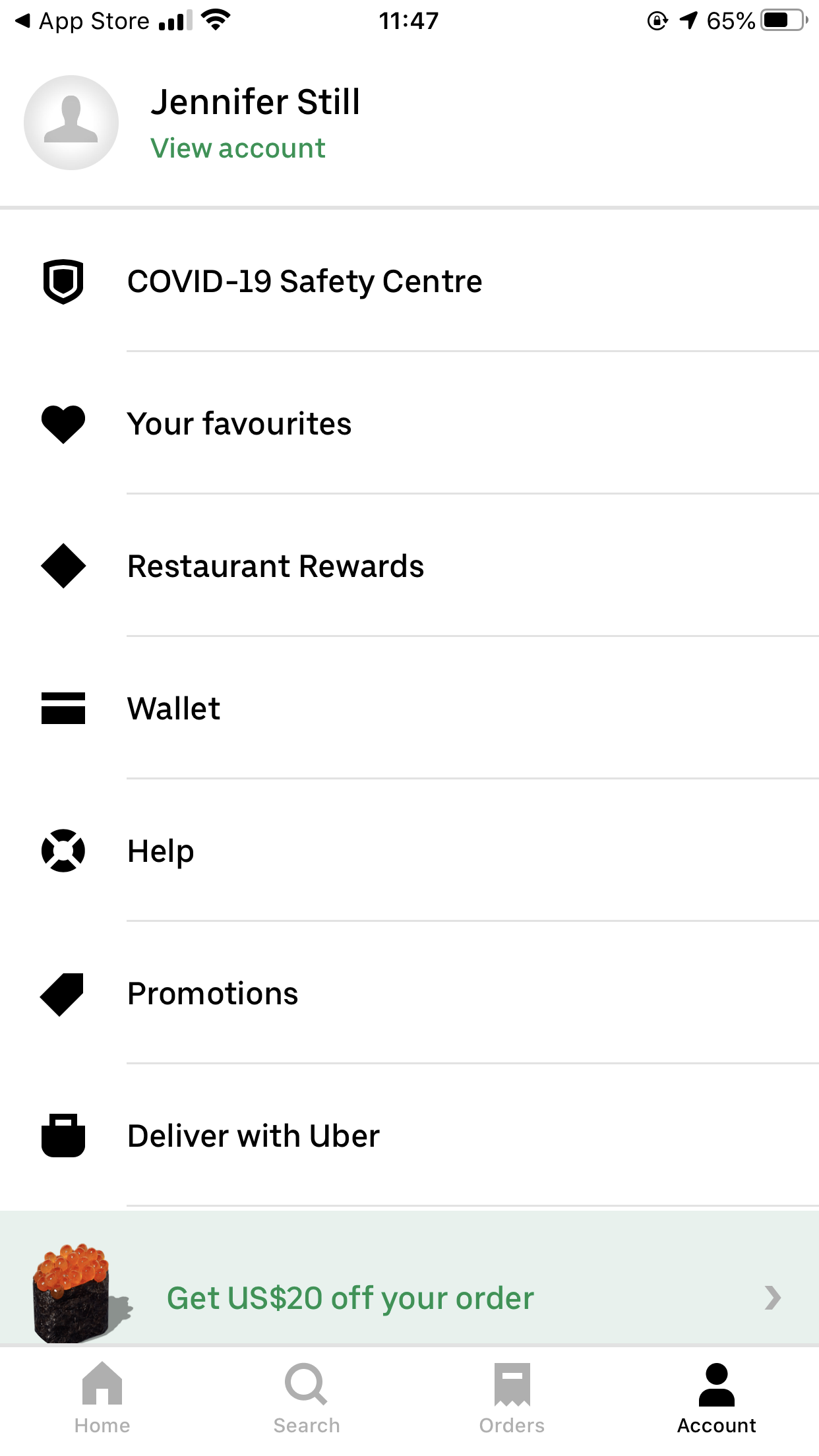The screenshot displays the App Store interface on a device with three out of four bars of data connectivity and Wi-Fi signal indicated as '1147.' The battery level stands at 65%. The account section reveals a user named Jennifer Steele who currently has a blank profile picture. Various features and sections are visible, including the COVID-19 Safety Center, Your Favorites, Restaurant Rewards, Wallet Help, and Uber Promotions. Notably, there's an offer for $20 off a future order. A small thumbnail shows a piece of seaweed adorned with orange fish eggs. At the bottom of the screen, the navigation menu includes options for Home, Search, Orders, and Account, with the Account tab highlighted in bold black letters.